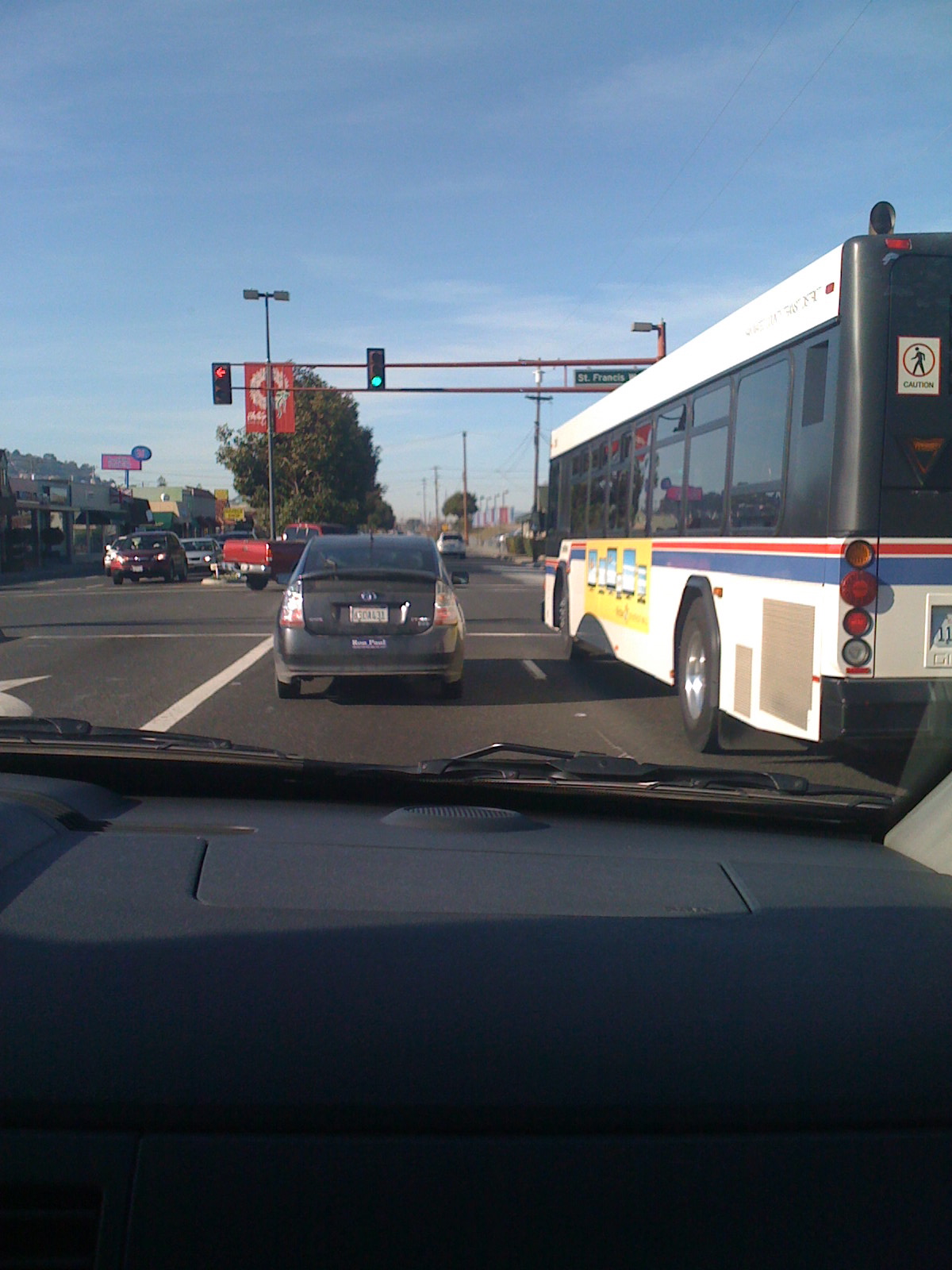An image depicts a clear blue sky with sparse white clouds. On the right side of the scene, a bus is visible, equipped with black-tinted windows and a white rectangular sign on its roof. The side of the bus features a combination of white and yellow panels, alongside a blue rectangle accentuated by a red stripe. At the rear of the bus, there is a red taillight, several other smaller lights, and a white caution sticker illustrating a pedestrian.

In the foreground, the camera captures the view from inside another vehicle, showcasing its dashboard and windshield wipers. A lamppost with a light on top and a traffic light are situated nearby; the green light is lit while the left signal glows red, indicating a lane closure or turn restriction. Additionally, there are various vehicles on the road, including a noticeable red truck. Lastly, a traffic sign with a red border and a blue circle on its top right corner can be seen in the scene.